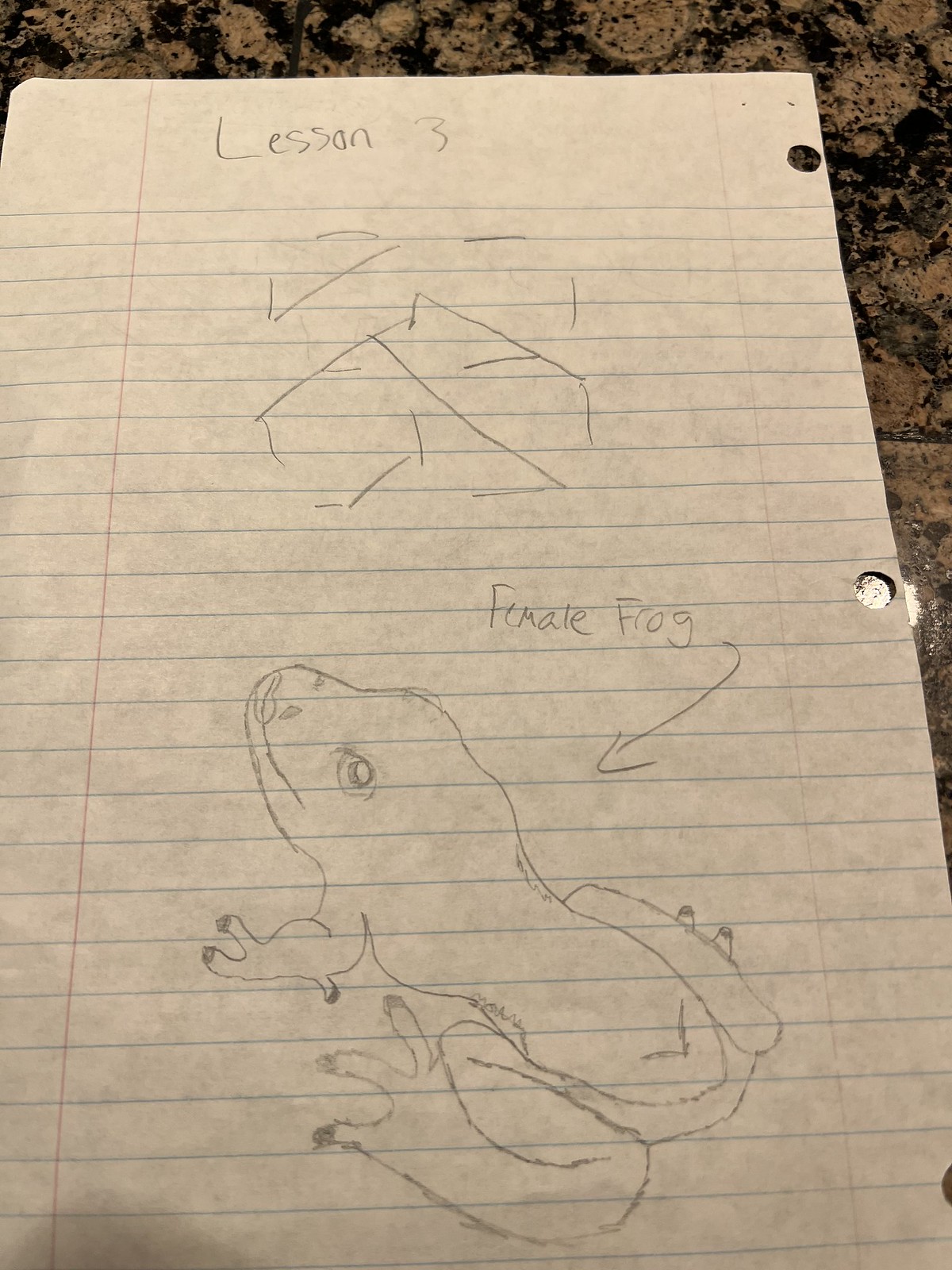On a piece of wide-ruled notebook paper, likely a child’s school notes, several pencil illustrations and writings are visible. The paper is oriented with the three binder holes along the right edge and is laid out on a brown and black marbled countertop. At the top of the page, “Lesson 3” is neatly written in pencil. Below this heading, there are various undecipherable line doodles scattered across the upper portion. 

The most prominent feature on the paper is located on the bottom half—a pencil drawing of a frog, labeled "Female Frog" with a downward-pointing arrow. The frog, characterized by its large, cartoonish eyes and lipstick-marked lips, is drawn with a left-facing head and body extending diagonally towards the bottom right corner of the page, resembling a tree frog. The reflection of an overhead light is visible through the middle binder hole, and a shadow cast by the person taking the photo is slightly discernible at the bottom of the image.